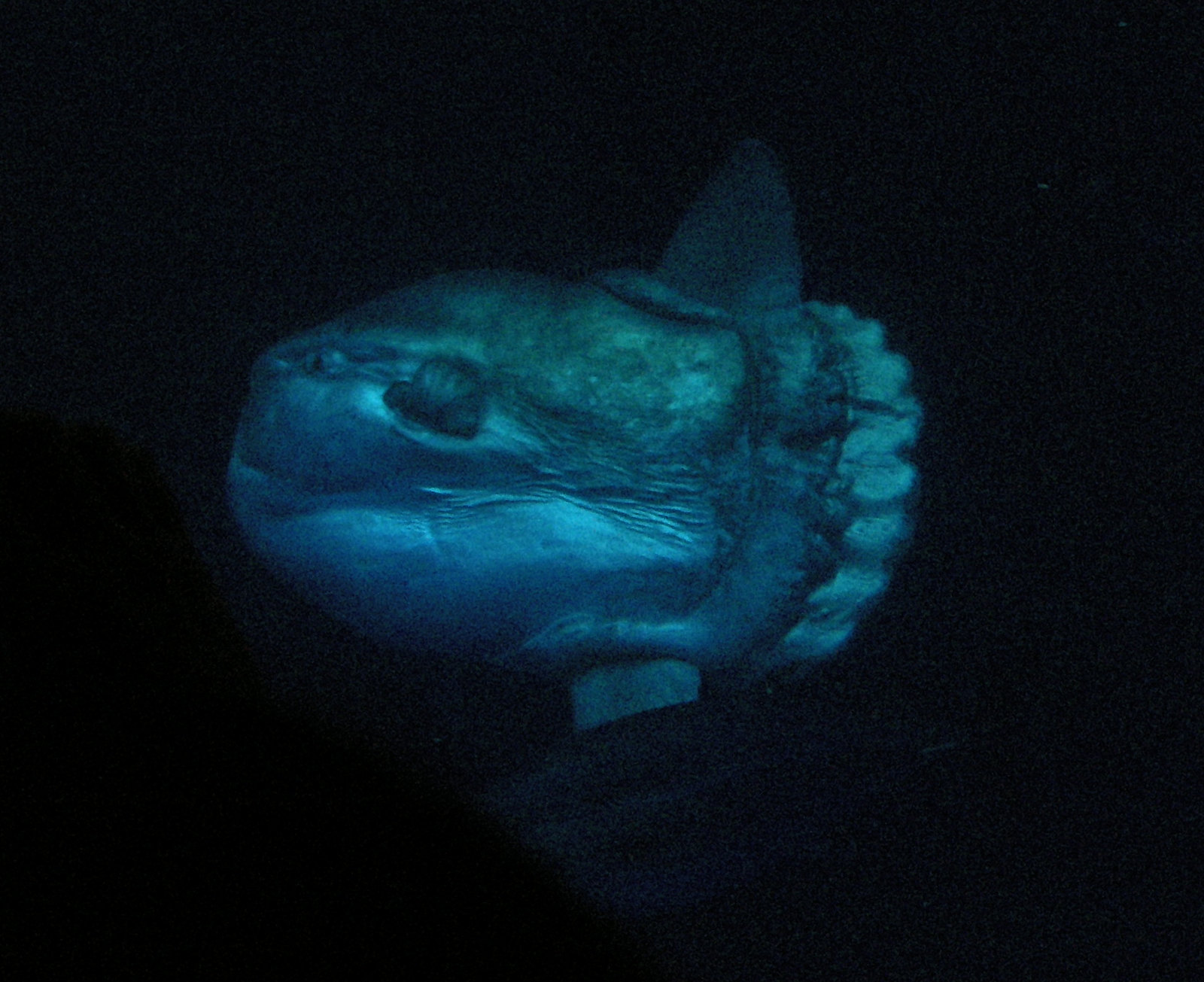The image showcases a luminescent blue-green sea creature with a notably misshapen and lumpy appearance, floating against a pitch-black background. The fish's unusual glow contrasts starkly with the dark surroundings, making its vibrant colors and unique form stand out. The fish features a round body characterized by numerous creases concentrated in its center. It appears to be missing one eye, replaced by a knot on its head, enhancing its eerie look. The fish has a single fin on the very top, a stubby ribbed fin at the back, another fin underneath, and a small fin at the front. The top portion of its body is mainly green fading into a silvery blue towards the bottom. This creature's glowing and misshapen form, set against the dark background, gives it an undeniably creepy and distinctive appearance.